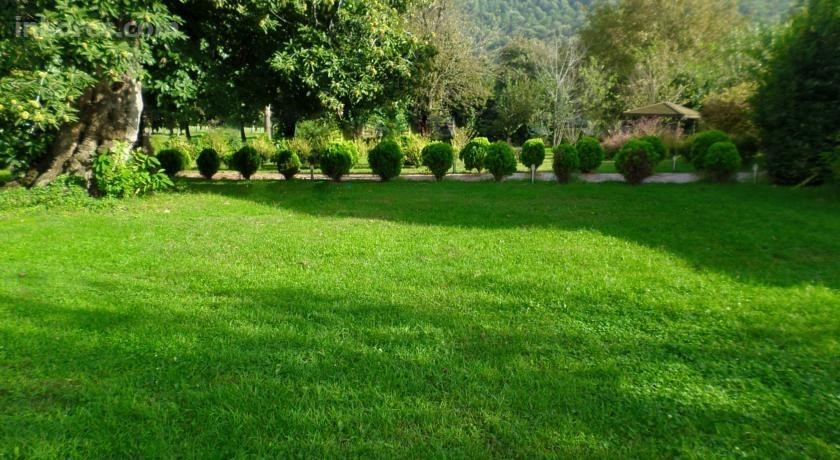This photograph captures a wide, neatly manicured green lawn that stretches across the lower half of the image, bathed in sunlight and interspersed with shadows cast by off-screen trees. The emerald lawn is partially shaded, suggesting a serene, sunny day. In the middle of the frame, a narrow, grey path, bordered by several small, round green bushes, cuts horizontally from right to left. On the left side of the image, a large, thick-trunked tree with an overhanging canopy provides substantial shade across the lawn and path. At the top-left, the dense branches of this tree arc gracefully over the walkway, adding a sense of scale and depth. In the hazy distance beyond the path, a cluster of more green grass and a traditional-style pagoda can be seen, nestled among more trees, adding an intricate focal point to this calm rural or park-like setting. The vibrant spectrum of colors, ranging from shades of green to earthy browns and hints of yellow, enhance the lush, vibrant feel of this picturesque outdoor scene.